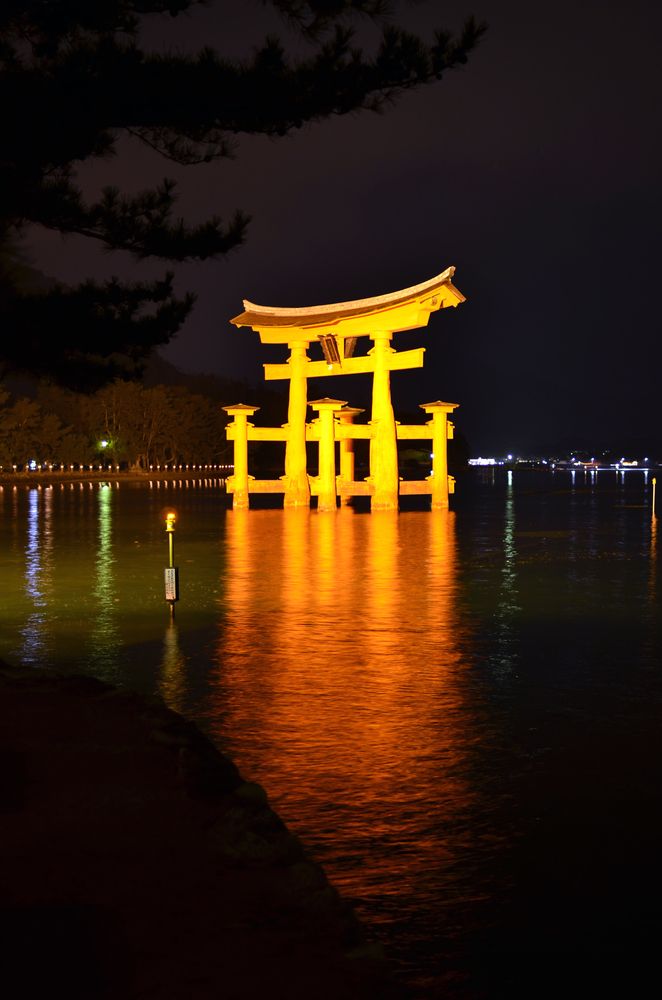This nighttime photograph captures an illuminated Japanese-style torii gate partially submerged in water. The torii gate, characterized by its classic horizontal crosspiece supported by vertical pillars, glows with a brilliant yellow light that reflects off the surrounding water, casting a shimmering orange glow. The scene is set against a backdrop of a dark, clear sky. On the upper left of the image, dark branches and leaves of a tree extend into view. In the background, a long bridge adorned with lights stretches across the water, leading towards a softly lit cityscape or village, adding depth to the scene. Additionally, a cylindrical post with Japanese characters, also lit by a small yellow light, is visible in the foreground, enhancing the cultural ambiance of the photograph.